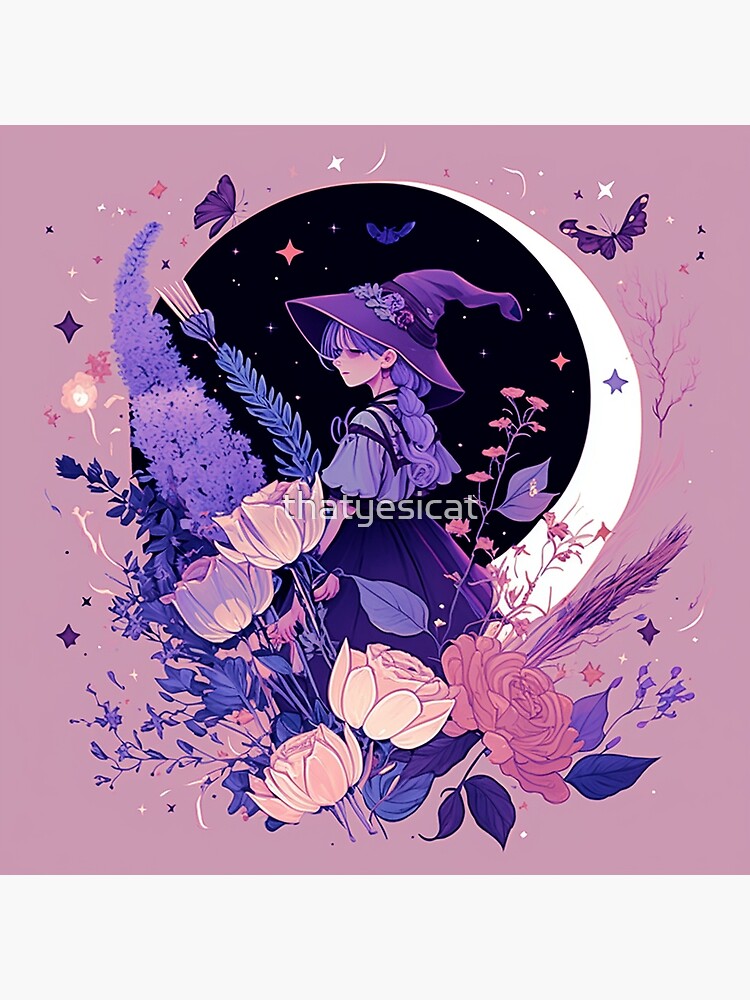The artwork portrays an enchanting anime-style young female witch, dressed in a period-inspired outfit consisting of a purple witch's hat, a light purple short-sleeve shirt, and a long purple skirt. Her long, flowing blue hair cascades down three-quarters of her back. She stands among an array of delicate flowers in varying shades of purple, pink, and red, with butterflies fluttering around her, particularly noticeable in the upper corners of the piece. The background features a dark night sky, which seamlessly transitions into a mystical eclipse, with white stars scattered across the blackened part of the sky and forming a crescent shape. The character's eyes are closed, suggesting she is lost in thought, creating a serene and contemplative mood. A discreet watermark reading "yes I can" is also present in the image.